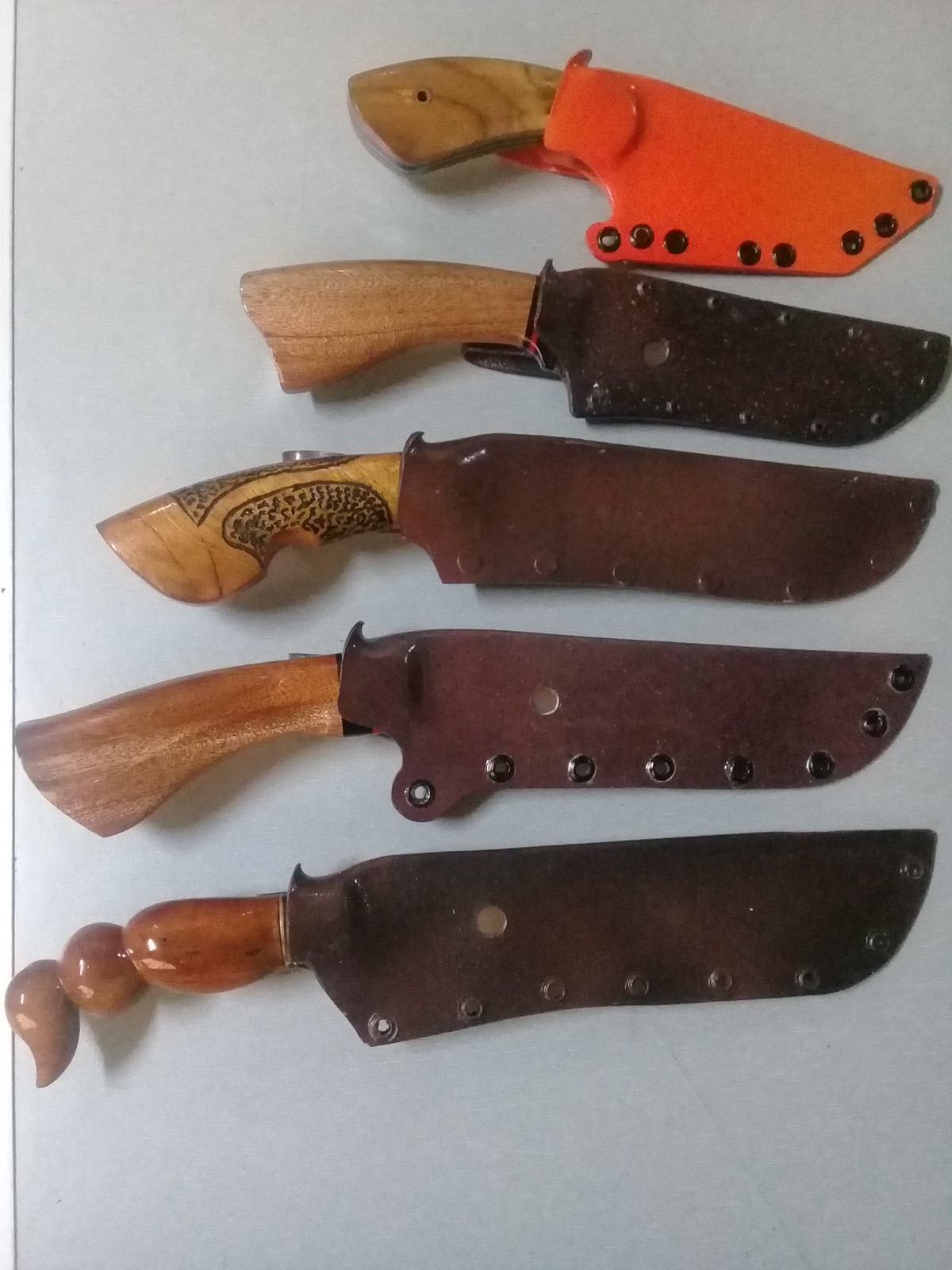This is a portrait-style photograph of a knife collection featuring five knives arranged in a vertical row from smallest at the top to largest at the bottom. Each knife is encased in a sheath with wooden handles visibly protruding. The smallest knife at the top has a bright orange sheath adorned with rivets. The remaining knives are housed in progressively larger brown leather sheaths. Notably, the second knife's sheath has an aged leather appearance, while the middle knife features decorative burnings on its handle. The largest knife at the bottom showcases a handle with three distinct sections, adding a decorative touch to the collection.